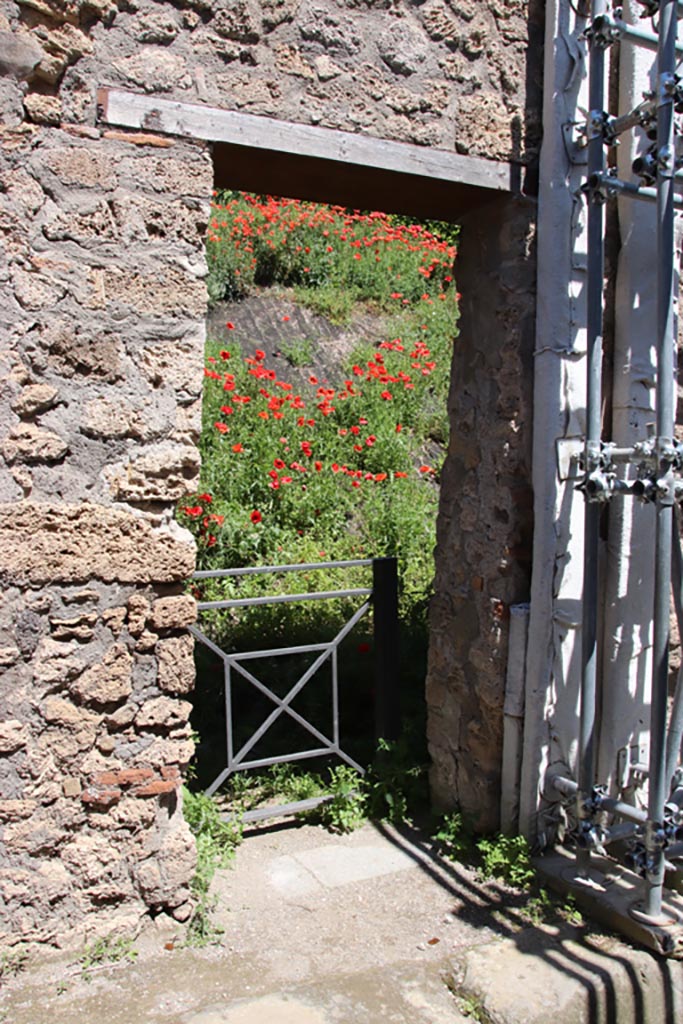In this rectangular photograph, we are presented with a serene garden entranceway bathed in bright sunlight. The composition features a stone wall, weathered with age, stretching from the lower left corner towards the center of the image, adorned with lush, cascading ivy. The ivy's vibrant green contrasts with the wall's ancient, gray stone, which bears patches of freshly reapplied white grout.

At the lower left, the back of a woman is visible from the waist up. Her blonde hair glows in the oversaturated light, and she is dressed in a light-colored tank top, revealing her bare arms. She is positioned facing the stone wall, her head gently angled downward, with her face obscured from view.

Adjacent to the woman is a rustic wooden gate framed by metal bars running vertically, blending seamlessly with the organic and historical ambiance of the entranceway. The right side of the image reveals a continuation of the aged stone wall, reinforcing the sense of an ancient, yet enduring, structure. The overall scene exudes a tranquil beauty, inviting the viewer to imagine the hidden garden beyond.